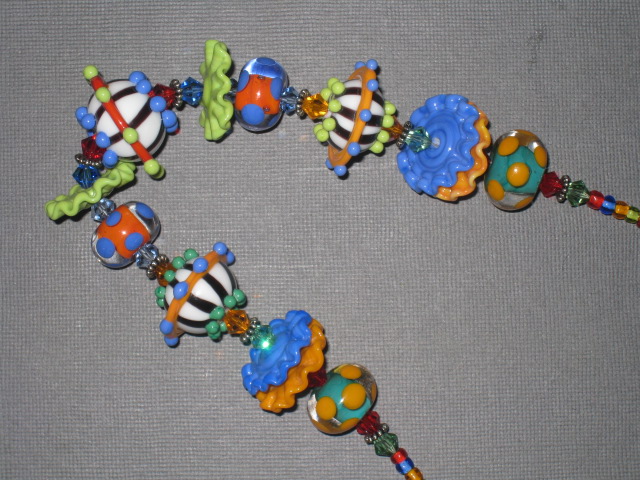This photograph showcases a highly detailed, colorful necklace, positioned on a gray fabric background. The necklace extends beyond the frame, suggesting its considerable length. It features an array of beads and decorative pieces of various shapes and colors, including blue, orange, green, and red. Symmetrically arranged, the beads and components include round, triangular, and oval shapes, as well as floral designs and metal dividers. Moving from the outer edges inward, the beads transition from simple multicolored beads to more intricate designs: an orange and green-brown piece, an orange and blue squiggly piece, and then a series of multicolored beads. Notably, there are ladybug-like pieces with wing-like designs, leading to a prominent central element. This centerpiece is round, white, adorned with four balls on each side, and capped with a red stick topped by four additional balls. The materials appear varied, with some beads looking like polished glass or acrylic, while others might be metal. The overall design, with its vibrant and eclectic mix of elements, suggests it could be a unique piece of jewelry, although its exact use remains ambiguous.